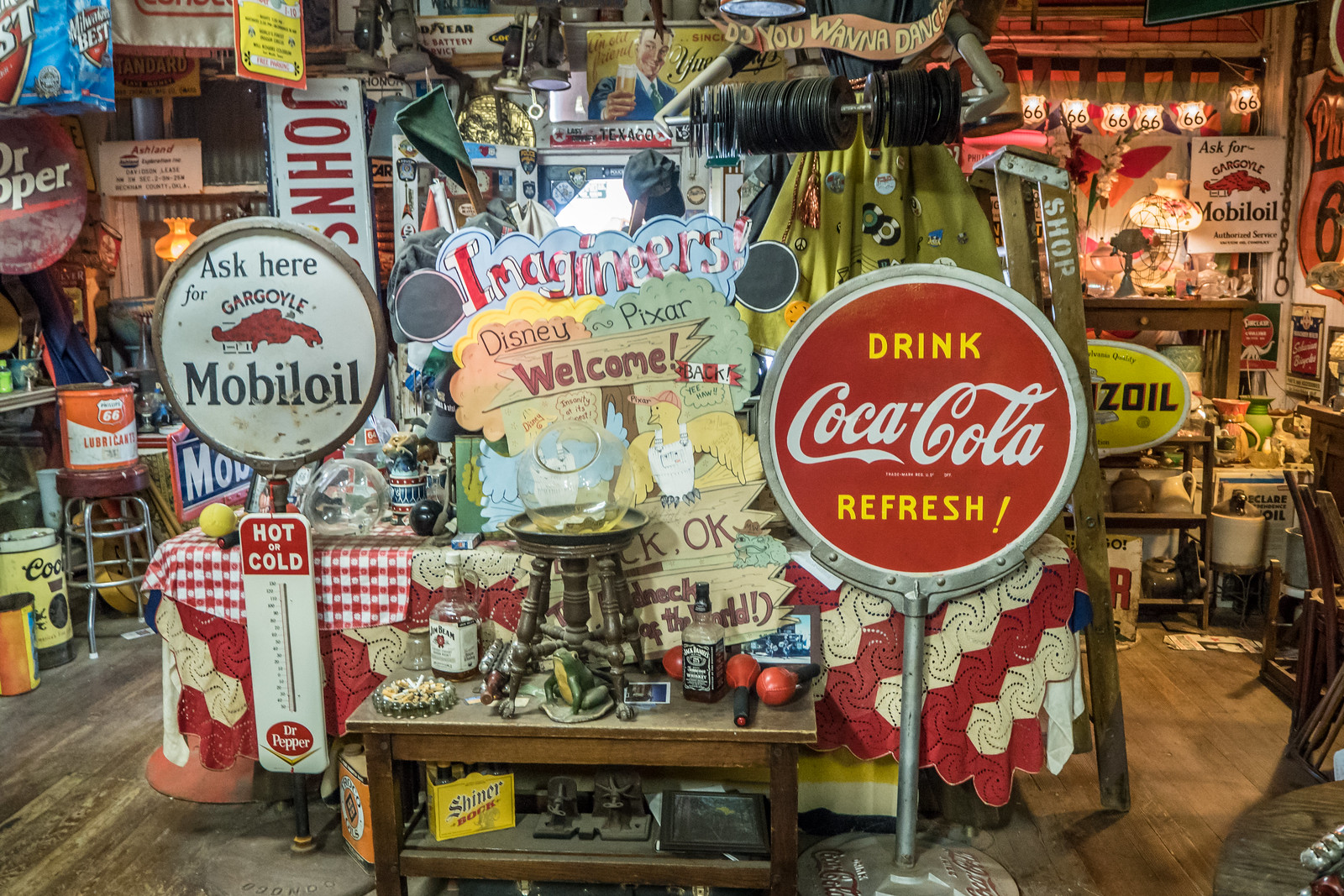This image captures a visually dense scene of a store display crammed with an eclectic mix of antiques and collectibles. In the center of the image, a notable blue rectangular sign with the word "Beginners" stands out prominently. Below this sign is a Disney Pixar Welcome sign, featuring a man drawn beneath the text and decorated in various colors, including red, green, and yellow. 

To the left of this central sign, there's an old advertising piece for Dr. Pepper. The vertical red and white sign has a header that reads “Hot and Cold” with a thermometer graphic below it; further down, "Dr. Pepper" is emblazoned in white against a red background. Adjacent to it, there is a round white gas globe that features the text "Ask Here," with an illustration of a gargoyle and the words "Gargoyle Mobil Oil." Above this gas globe, an older sign with the name "John" in red font on a white background is visible.

On the right side of the Disney Pixar sign, an eye-catching circular Coca-Cola sign dominates the scene. This sign has a red background with the word "Drink" at the top and "Refresh" at the bottom, both in yellow font, while the central text "Coca-Cola" is in white. 

The background and surrounding areas of the image are filled with a plethora of other vintage items, including shelves stacked with various goods, an old Jack Daniels whiskey bottle, maracas, a Coors ice chest, and an old Pennzoil sign. Old vinyl records are neatly lined up on a metal pole, enhancing the nostalgic atmosphere. The scene is set against a backdrop of aged wooden flooring, adding to the rustic, treasure-trove ambiance of the store.